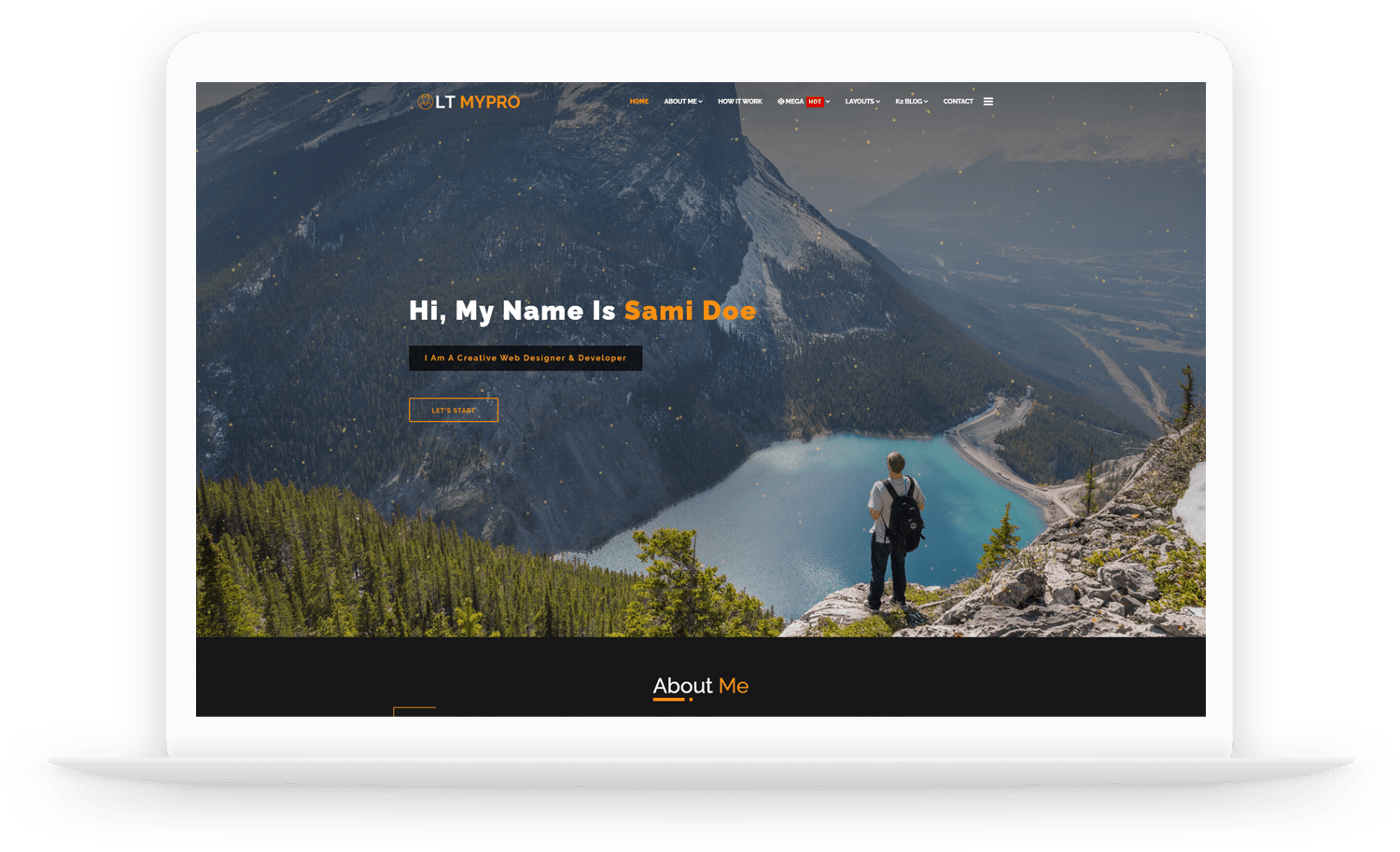**Descriptive Caption:**

This screen capture showcases a personal web page of a creative web designer and developer. In the upper left corner, the page features the logo 'LT my pro'. The main navigation tabs are spread across the ribbon at the top, though the font is too small to read clearly. Central to the page, a welcoming text is displayed saying "Hi, my name is S-A-M-I-D-O-E" — with 'Hi, my name is' in white text and 'S-A-M-I-D-O-E' in striking orange. Beneath this text, within a black rectangular banner, it states "I’m a creative web designer and developer."

The background image is a breathtaking landscape captured from a high mountain peak. It overlooks a serene lake nestled between mountains. Positioned on the right edge of the cliff within the image is a person clad in a gray shirt, black pants, and a backpack, presumably representing the site owner, SAMIDOE.

At the bottom section of the page, in white lettering, is a heading that reads "About Me," with 'Me' highlighted in orange. This layout suggests that this web page likely serves as a personal portfolio for the web designer and developer, targeting prospective employers or clients.